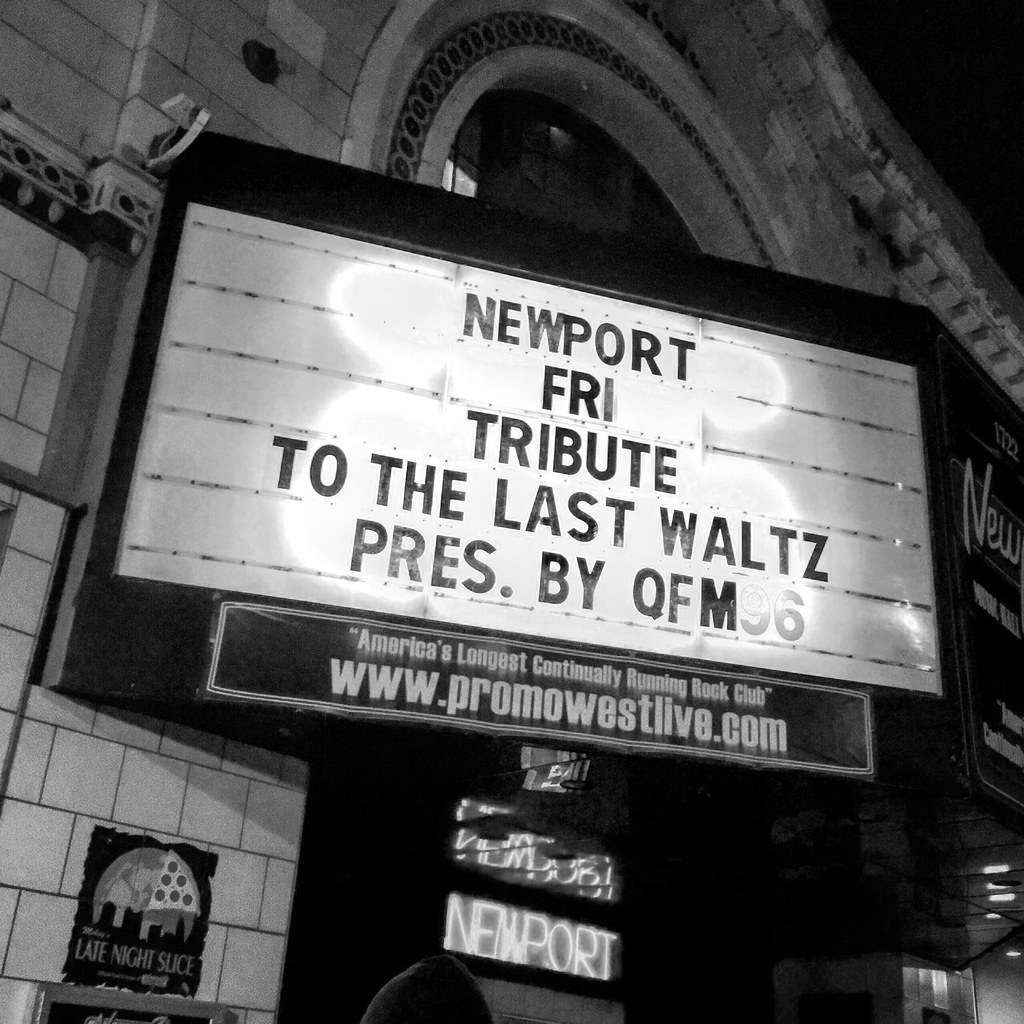The image depicts an outdoor nighttime scene of a historic stone or brick building, featuring a large, brightly lit movie theater marquee with neon lights. The marquee prominently displays the text: "Newport Friday Tribute to The Last Waltz, Presented by QFM 96." Below the marquee, a black rectangular sign reads: "America's Largest Continually Running Rock Club www.promowestlive.com." Additionally, there's a smaller poster on the wall below these signs that advertises "Late Night Slice," with an image of half a pizza. The perspective of the photograph is from ground level, looking up at the illuminated marquee and the building's arch, emphasizing the grandeur and historic charm of this American club. There are no people visible in the image, further focusing attention on the marquee and the architecture. The scene is set against a dark night sky.